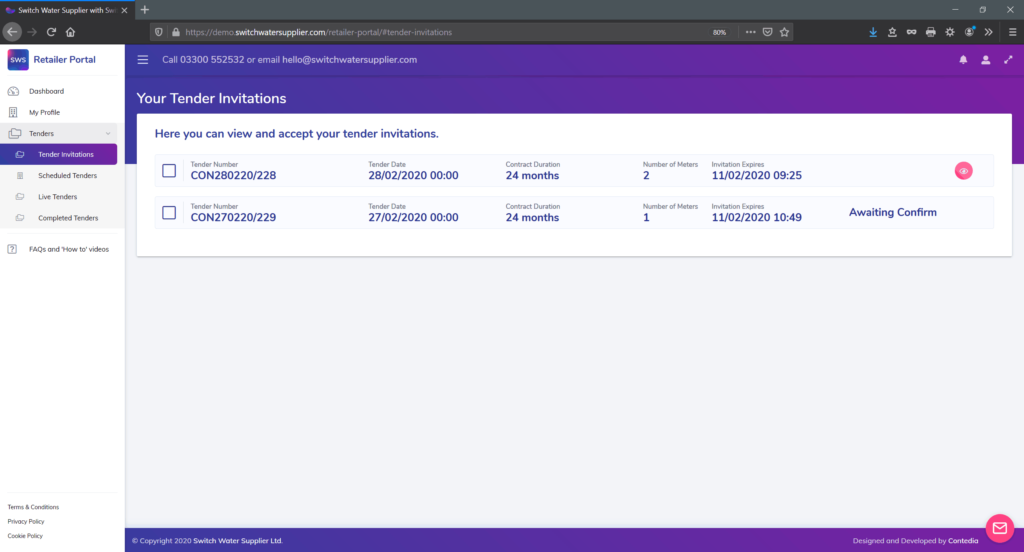At the top of the image, there is a large gray header. Towards the left, a browser tab is open with a black background displaying the text "Switch water supplier with S…" which is cut off. Below the header, there is a black navigation bar featuring a circular gray icon indicating a back button. To the right of this icon, there is a disabled forward button, not highlighted to show it is inactive. Adjacent to the forward button is a white refresh button. Further right, there is an icon of a house outlined in white.

The address bar, positioned next, is a medium gray fading into a dark violet ombre on the left background, transitioning into a vibrant light violet on the right. In the address bar, a white dropdown menu is visible featuring three horizontal lines beside the text "call 03300 552532, or email hello@switchwatersupplier.com."

Below the address bar, a dividing line separates the sections. The next segment contains the text “Your Tender Invitations” in white. Underneath, there is a long rectangular section with a white background. It begins with the instruction, "Here you can view and accept your tender invitations," written in dark purple. The section features two listings, both with tick boxes on the left against a light gray background. Each listing includes details:

- The first listing shows:
  - Transfer Number: CON280220/228 in dark blue
  - Tender Date: 28/02/2020 00:00
  - Contract Duration: 24 months
  - Number of Meters: 2